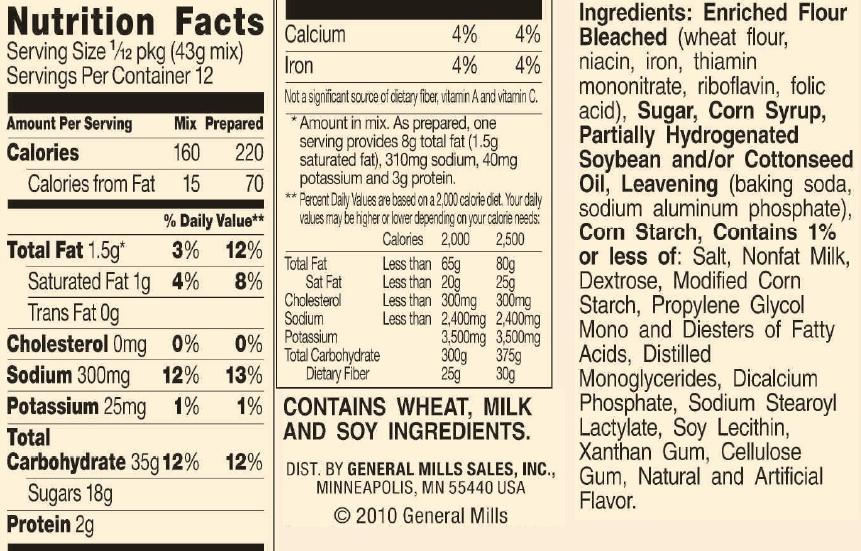The image depicts the nutrition facts label of a packaged food item produced by General Mills. The package contains 12 servings, with each serving size being approximately 43 grams. The caloric content per serving is 160 calories, while the prepared caloric value is listed as 220 calories, indicative of additional ingredients such as milk or sugar being added for consumption.

The ingredients list includes enriched bleached flour, sugar, corn syrup, and partially hydrogenated soybean and cottonseed oil, and it contains wheat, milk, and soy ingredients. General Mills Sales, based in Minneapolis, Minnesota, distributed this product in 2010. The background color of the label is a light yellow, off-white hue. Given the nature of the ingredients, the serving size descriptions, and the association with General Mills, it suggests that the product is a type of cereal.